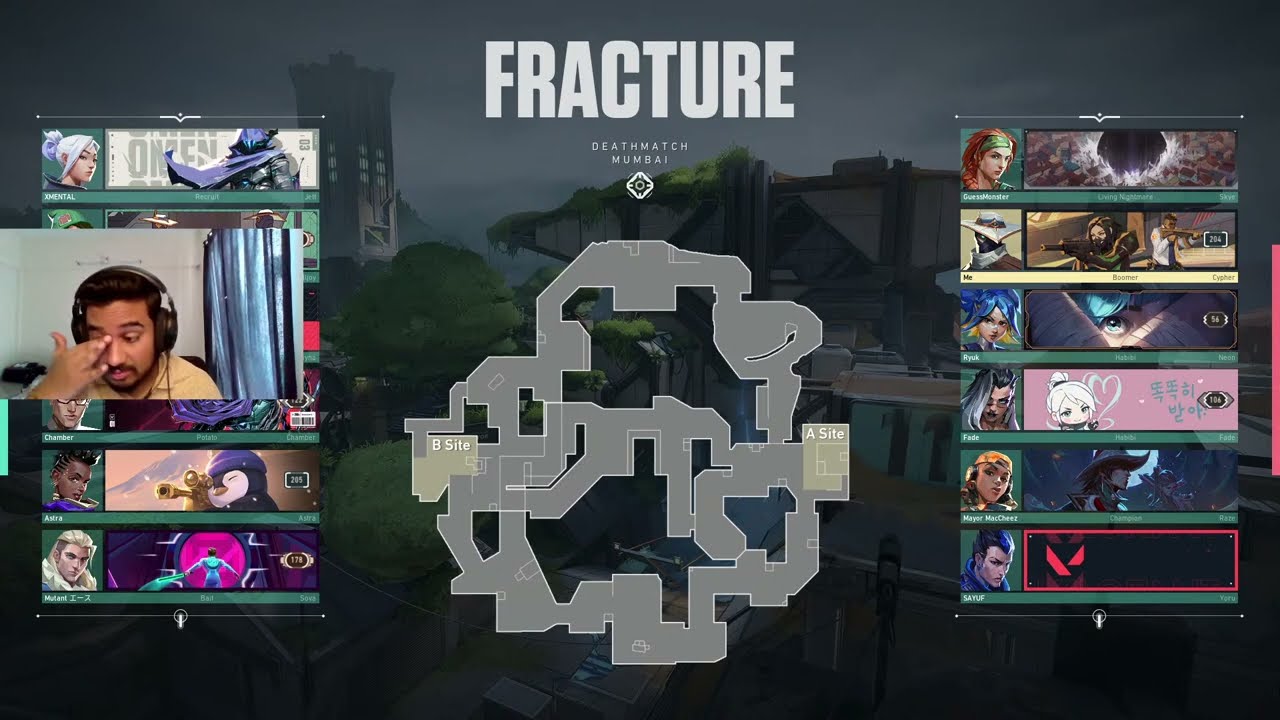The image depicts a screenshot from the video game "Fracture," specifically set in the "Deathmatch Mumbai" mode, as indicated by the bold, all-caps text at the top of the image. The central focus is a detailed blueprint map, showing labeled "B Site" and "A Site" areas, connected by a series of tunnels, depicted in light beige against a gray background. 

Flanking the map on both sides are character panels featuring various anime-style avatars, including a lady with a green headband, a person with blue hair, a girl with white and grey hair, a blonde-haired girl, and a character with a bun, among others. These represent different playable characters in the game.

On the left side of the image is a live video feed of the streamer, a young man of Southeast Asian descent. He is wearing a light mustard-colored or beige shirt, headphones, and has dark brown hair and a short brown beard. He is rubbing his left eye, with a blue curtain visible behind him and a white wall to his right.

In the background of the game map, there is a dark cityscape dotted with green trees and interconnected buildings resembling obstacle courses, adding a layer of depth to the gaming environment.